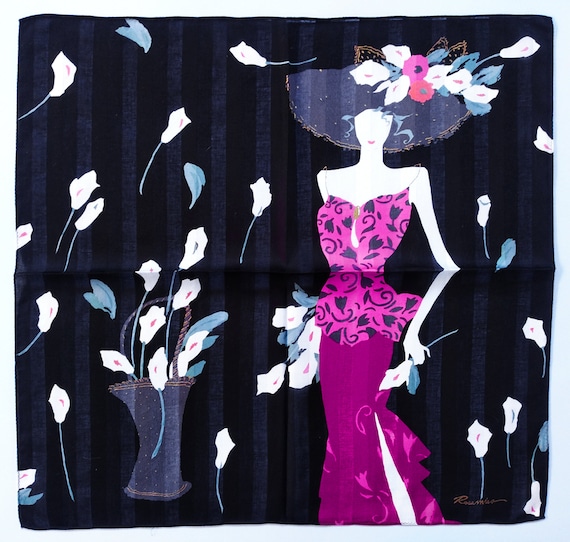The image is a highly detailed painting on what appears to be pleated or striped fabric, with a sophisticated interplay of hues giving a creased effect akin to an opened handkerchief. Framed by a narrow pale blue border, the dark blue and black stripes form a striking background. Central to the composition is the figure of a slender, tall woman with pale skin. She dons a long fuchsia skirt with a slit, embellished with floral designs near the bottom, and a vibrant peplum-style top in hot pink adorned with black flowers. Her accessories include a broad-brimmed black hat, lavishly decorated with a bow and an array of flowers—white calla lilies, and a mix of various colorful blooms like pink and red flowers. Below her, possibly stitched onto the fabric, is a denim-colored basket filled with calla lilies, appearing as if some are floating freely around her. In her right hand, she holds a bunch of these lilies, while a single calla lily graces her left hand. The artist's long golden signature, beginning with an "R" (resembling "Erasmuson"), is elegantly inscribed at the bottom right, completing this captivating fabric artwork.